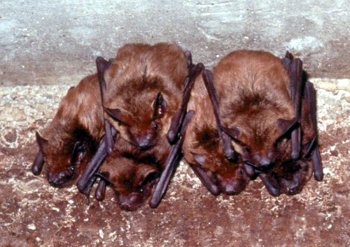This is a detailed color photo close-up of a group of six bats huddled together in a pyramid formation on the ground, which appears to be old cement, possibly in a garage with a solid concrete wall in the background. The bats have brown fur-like bodies with dark brown, tucked-in wings, and small, sharp-pointed ears. Their eyes appear to be closed, indicating they are sleeping. The bats form a layered pile, with two on the bottom and additional ones on top, creating a clustered, entangled appearance. Overall, they present as a singular, cohesive mass of brown bodies and folded wings, lying on what might be a rock or a similar earthy surface.